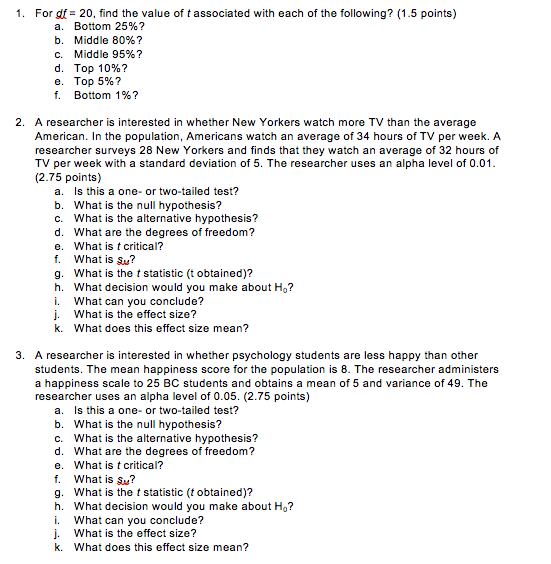In the image, there is an extensive amount of text organized in a structured format. 

In the top left corner, there's a large, bold "1." To the right of this number, the text poses a question that reads: "For df = 20, find the value of t associated with each of the following?" To the right of this query, it is noted as being worth "1.5 points." 

Following this text, a list labeled from "a" to "f" is presented, each with specific percentile information:
- a) Bottom 25%
- b) Middle 80%
- c) Middle 95%
- d) Top 10%
- e) Top 5%
- f) 1%

Below this list is the second question, marked with a bold "2." It states: "A researcher is interested in whether New Yorkers watch more TV than the average American in the population. Americans watch an average of 34 hours of TV per week. A researcher surveys 28 New Yorkers and finds that they watch an average of 32 hours of TV per week with a standard deviation of 5. The researcher uses an alpha level of 0.01." The section is noted as "2.75 points," and this question also has sub-questions labeled from "a" to "k."

The third question is located towards the bottom middle of the image, labeled with a large "3." It states: "A researcher is interested in whether psychology students are less happy than other students. The overall happiness score for the population is 8." This section, like the previous one, is followed by sub-questions labeled from "a" to "k."

The image is densely packed with text that appears to be part of an exam or assignment focused on statistical analysis and hypothesis testing.